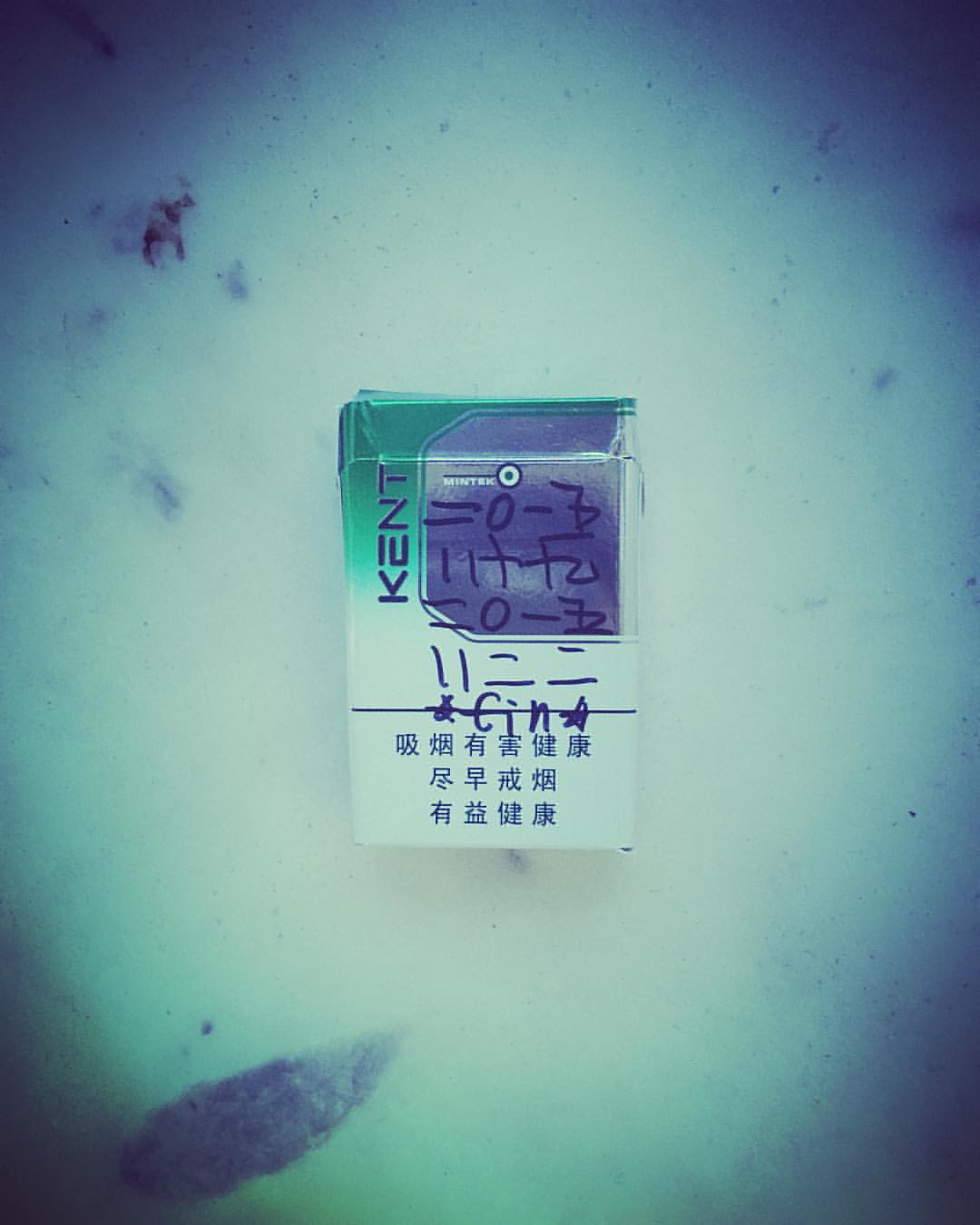The image depicts a box resembling a cigarette package, featuring predominantly Asian writing, which appears to be Chinese, that is unreadable to the viewer. The upper section of the package is a vibrant green, transitioning to a white shaded area at the bottom. A distinctive purple or blue section is located near the top. There are black lines and circular markings, presumably made with a magic marker, across the midsection. Additionally, on the side of the package, the word "KENT" is printed diagonally. The box is situated on a dirty surface covered with black marks and brown strings, contrasted by a white background.